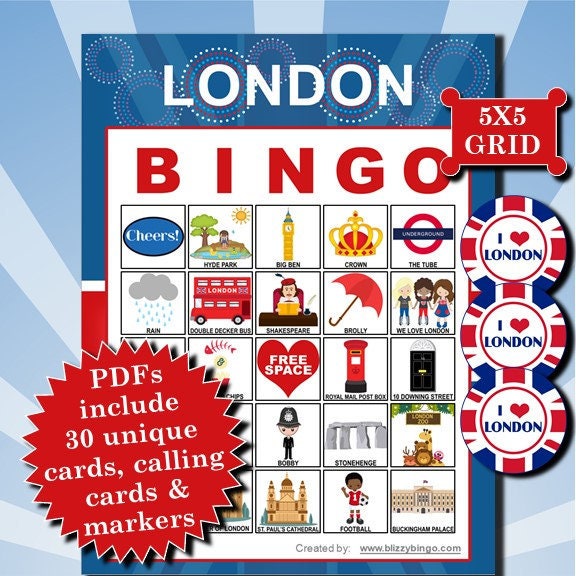The image is a square advertisement for a group of PDFs called "London Bingo." It features a light blue background with blue stripes, superimposed with a bingo card. This card has a white 5x5 grid with "BINGO" written in bold red letters at the top. Each cell of the grid includes icons and text representing unique British and London-related landmarks and symbols, such as Big Ben, the Tube, a crown, Hyde Park, Stonehenge, and the phrase "Cheers." The right side of the image is adorned with three circular badges displaying the Union Jack and the phrase "I ♥ London." In the bottom left corner, a red star medallion indicates that the PDFs include 30 unique cards, calling cards, and markers. The advertisement is primarily decorated in red, white, and blue tones, corresponding with the colors of the British flag. The text also highlights that the bingo game involves spotting these icons and marking them off, with a win achieved by completing a row, column, or diagonal.